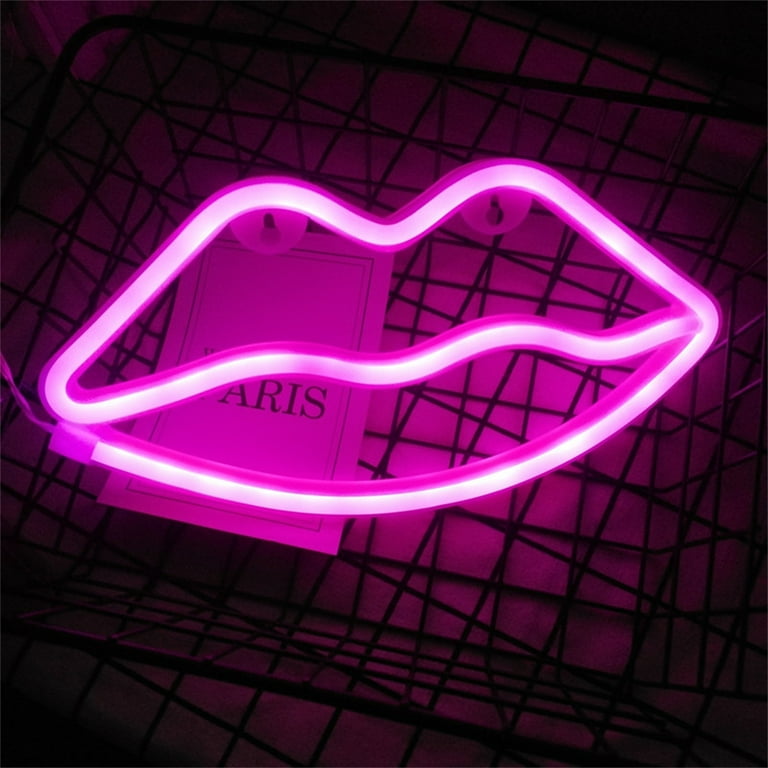The image depicts a vibrant neon sign shaped like a pair of closed lips, emanating a pink to fuchsia glow. The neon sign, resembling lips with lipstick, illuminates the entire scene with its vivid light. Below the lips, on the left side, there's a handle-like structure extending out, and a small rope is attached to it. The sign is housed within a black, metal-like basket or grate, resembling a metal dog cage. Behind the sign, a piece of paper with partially obscured text reads "Paris," with the "P" cut off. The setup includes other structures that appear to be metallic gratings or similar gates, which frame and support the sign.